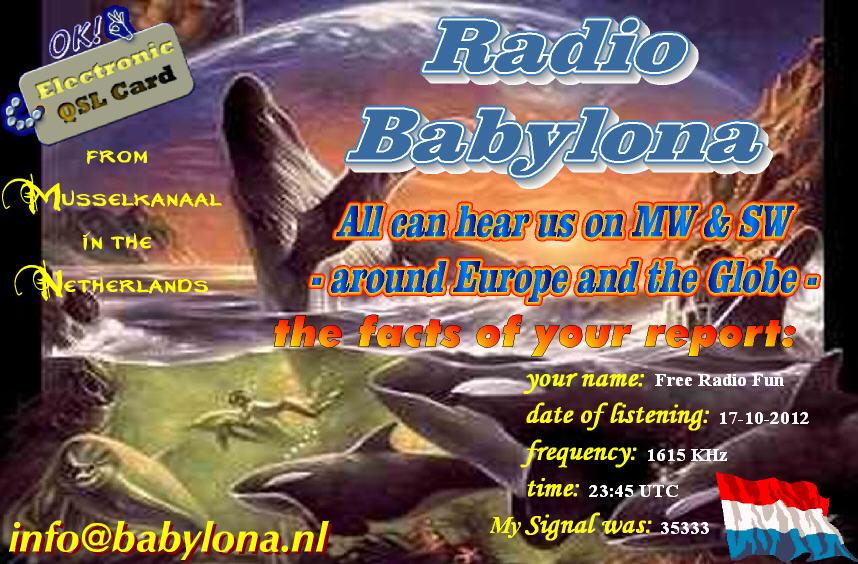The image is an advertisement card for "Radio Babylonia," featuring a detailed fantasy background that depicts an ocean scene filled with various sea creatures, such as whales, sharks, and large turtles. Above the ocean, there's a rock formation and a large planet visible in the sky, adding to the fantastical ambiance. 

In the upper right corner, the title "Radio Babylonia" is displayed prominently in large blue letters. Below this, in a darker blue font, is the text: "All can hear us on MW and SW around Europe and the globe." This text is highlighted in orange. Further down, in orange, it states: "The facts of your report." The card collects technical and listening details including: "Your name, free radio fun, date of listening: 17-10-2012, frequency: 1615 kHz, time: 2345 UTC, and signal: 35333." 

In the top left corner, there is an "OK" hand symbol beside a card that reads, "Electronic SL card." Adjacent to this, in yellow text, it says, "From Mussel Canal (Musselkanaal), the Netherlands." The lower left corner includes the contact email: "info at babylonia.nl."

A national flag with red at the top, white in the middle, and blue at the bottom is displayed alongside the other elements. The overall composition blends the technical details of the radio broadcast with an imaginative, aquatic theme.